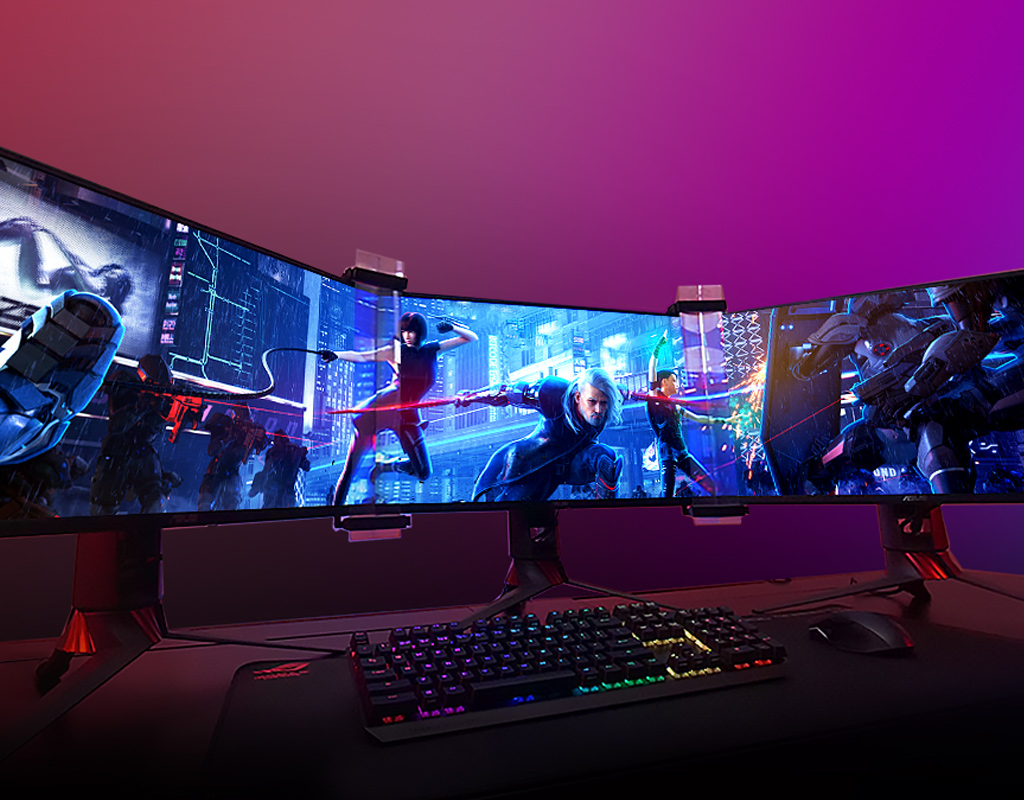In this photograph, we see an elaborate gaming setup within an office, featuring a striking three-monitor display. Each wide-screen monitor is interconnected, creating an immersive experience for the user. The screens collectively showcase a dynamic 3D video game, depicting futuristic characters engaged in combat, wielding swords, and utilizing whips against robots in a high-tech cityscape. The backdrop of the scene is enriched by a vibrant pink and purple-lit wall that complements the desk's matching color scheme. 

In front of the screens sits a rainbow-hued backlit keyboard, displaying a spectrum of colors from purple on the left to blue, green, yellow, and red towards the right side. Accompanying the keyboard is a black mouse positioned to the right. Additional gaming peripherals, including two handheld controllers, are discernible in the shadows to the right of the keyboard, enhancing the overall advanced gaming ambiance.